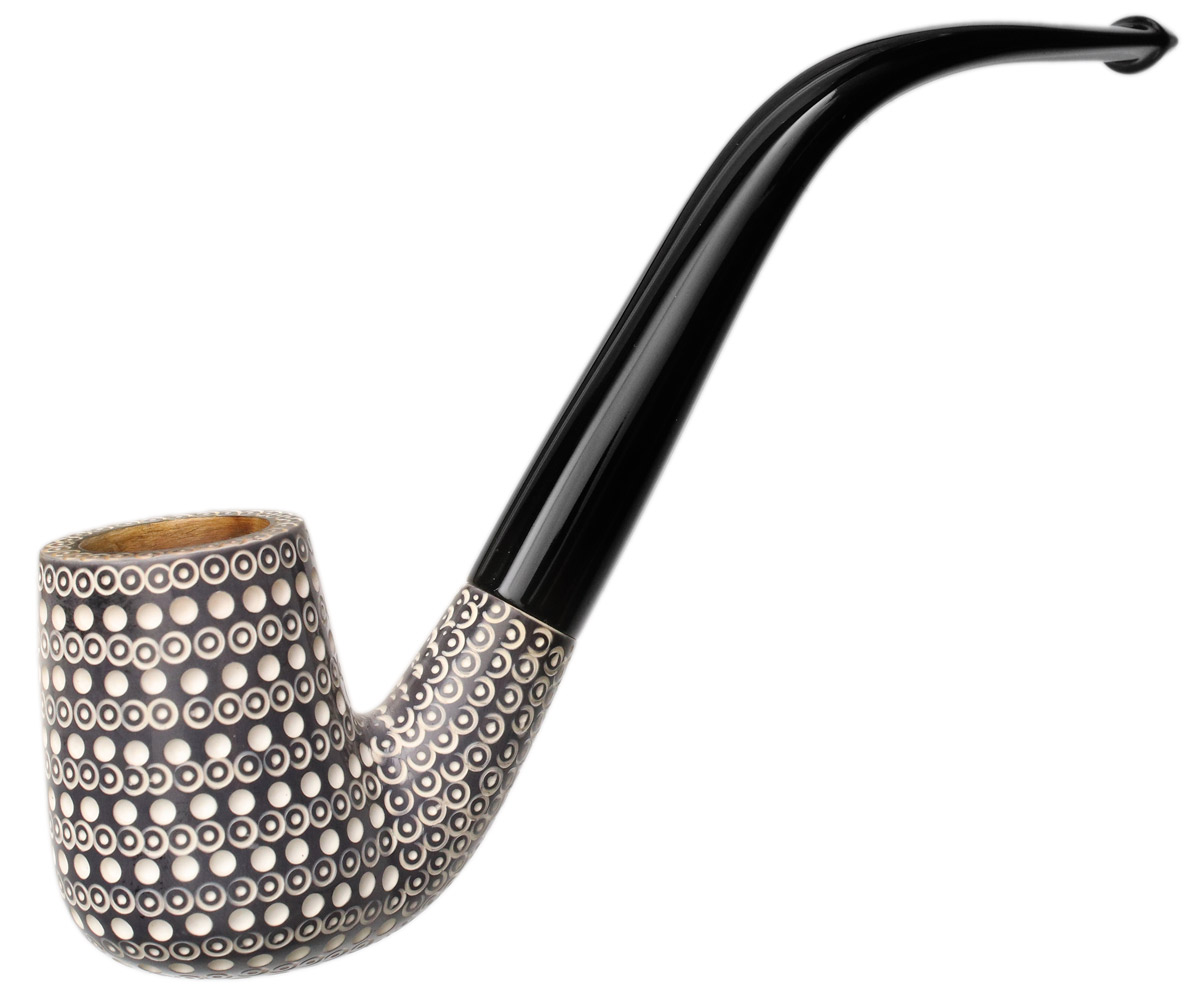The image features a meticulously crafted smoker's pipe, staged against a solid white background with artificial lighting that accentuates its fine details. The pipe's handle is a sleek, solid black that curves elegantly from the mouthpiece, which is contoured and polished to reflect light in a narrow line down its center. As the handle transitions, it becomes decorated with a distinctive circular pattern, featuring larger solid circles interspersed with circles containing smaller white dots, creating a visually appealing repeating motif.

At the base of the handle lies the bowl, designed for holding tobacco. This section is distinctively wooden with a rich light brown hue, contrasting beautifully with the pipe's otherwise monochromatic theme. The bowl's exterior bears the same intricate design as the handle, with the larger circles giving way to circles containing white dots as they ascend. The pipe as a whole presents a sophisticated blend of black, gray, and white, making it a striking piece likely intended for display or sale on platforms like eBay or Etsy. This detailed, full-color photograph captures the pipe's elegant and intricate craftsmanship, reflected in every etched and painted detail.